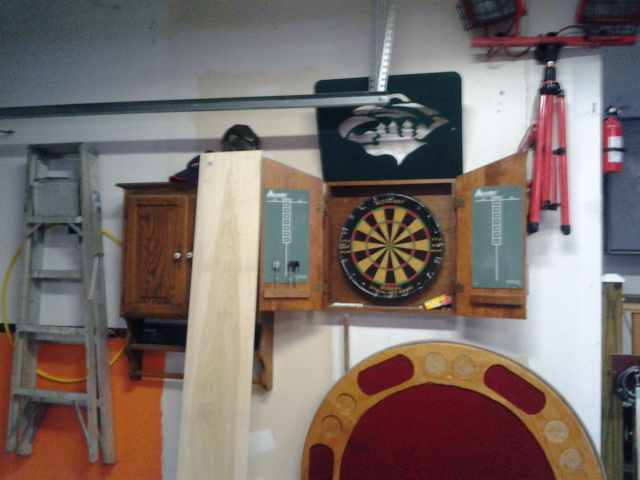The photograph, though blurry, captures the interior of a garage featuring a variety of items and structures. The walls, primarily painted white but with visible patchiness and beige areas, support various hanging items. Dominating the scene is a dartboard framed by a large orangey wood cupboard with green scoreboards on either side and a white T-shaped score structure in the center. Just beneath it lies a round, red velvet-covered poker table, propped against the wall. 

Surrounding these focal points, a fire extinguisher is mounted on the wall, alongside a wooden cabinet. A wooden board rests against this cabinet near the dartboard. In another section, an aluminum metal structure, possibly the garage door track, hangs down. Adjacent to this, a small orange square, potentially paint or a notice board, is visible. Additional items such as a metal ladder and a hula hoop are also hung on the walls, contributing to the cluttered yet intriguing interior of the garage.